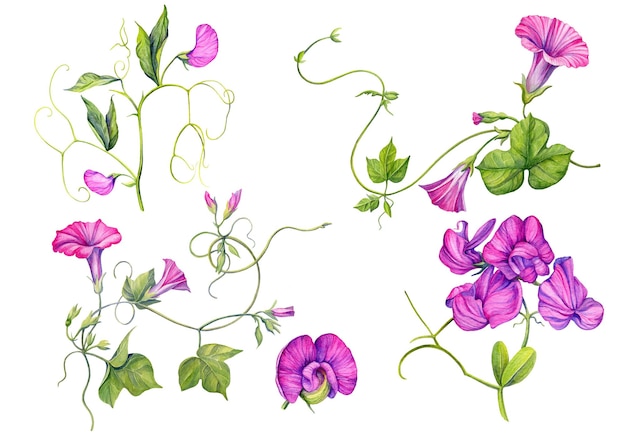This detailed image showcases a vibrant, lifelike drawing of purple-pinkish, trumpet-like flowers with lush green leaves set against a stark white background. The flowers, resembling smaller petunias or bell-shaped blooms, appear in various stages of blooming. They are depicted on long, spiraling, and vine-like stems, some solid and others delicate, lacy tendrils that wrap around and intertwine intricately. Notably, some stems feature clusters of three round-pointed leaves, while others taper off into curling spirals without flowers or leaves. These vividly drawn flowers, which often attract hummingbirds, stand out against the white backdrop, emphasizing their intricate details and natural beauty.